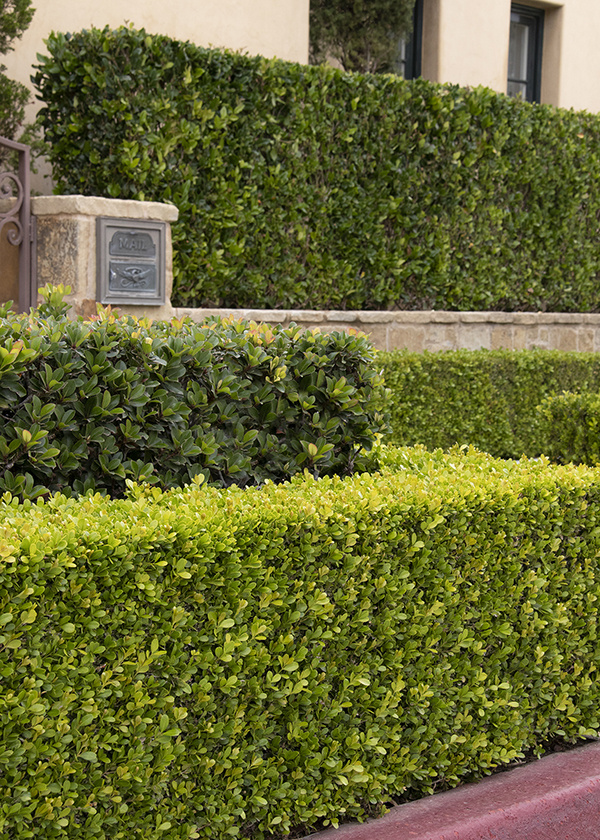The full-color photograph, taken outdoors during the day using natural light, captures a vertically rectangular scene devoid of any people, animals, or watermarks. The focal point of the image is a well-maintained array of boxwood trees and hedges, varying in height and color, that line a beige stone edifice. In the foreground, the boxwoods appear lighter green, while those in the background have darker, more robust leaves. The composition includes several distinct elements: a black mailbox with the word "mail" on it, a gray metal door, an iron gate, and black windows on a brown building visible in the background. To the lower right, the curb of a sidewalk or road made of gray concrete is visible. A plaque on the stone wall and the iron fence in the upper left corner add further detail to the setting, suggesting this is the landscaped entrance to a home. The angle of the shot, taken from a side perspective, emphasizes the vibrant greenery and the architectural features of the area.